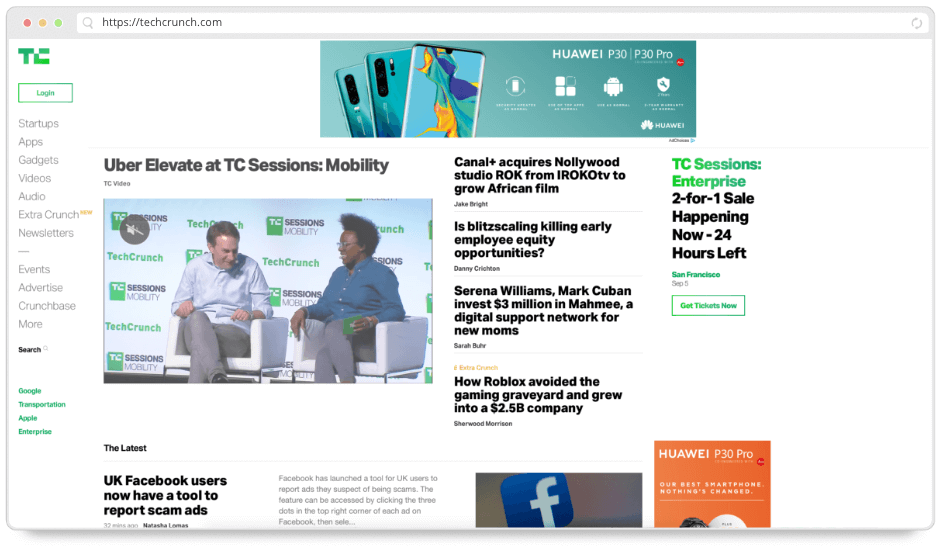The homepage of TechCrunch.com features a dynamic and bustling layout. At the top, there is a prominent advertisement by the notable Chinese tech giant, Huawei, showcasing their latest products. Below, the lead story centers on "Uber Elevated" as part of the TC Sessions: Mobility series, highlighting a recent conference presented by TechCrunch. The accompanying image depicts a lively discussion between a white man with short black hair dressed in a blue dress shirt and gray pants, and a black woman with a frizzy afro hairstyle, also in a dark blue dress shirt and gray pants, seated on couches against a backdrop themed for Sessions Mobility.

To the right, several of the day's top stories are listed:
1. "Canal Acquiring Fabled Hollywood Studio, ROK" - with a focus on expanding African film.
2. "Is Blitzscaling Killing Early Employee Equity Opportunities?" - an in-depth, issue-oriented analysis.
3. "Serena Williams and Mark Cuban Invest $3 Million in MAMI" - detailing the support for a digital network for new mothers.
4. "How Roblox Avoided the Gaming Graveyard and Grew into a $2.5 Billion Company" - exploring the company's significant growth.

Towards the bottom of the list, one can find a snippet of another article about a new tool for UK Facebook users to report scam ads. Below this is a section filled with more advertisements, including another from Huawei, this time promoting their P30 Pro in a small, orange rectangular box.

In the right-hand column, there's an announcement in TechCrunch's signature green font about the TC Sessions: Enterprise event with a two-for-one sale happening for the next 24 hours. 

On the extreme left-hand side of the page, navigation options are available, offering categories such as startups, apps, gadgets, video, and audio links. There's also something called "Extra Crunch," presumably a premium membership feature offering exclusive content. The lower section contains links for events, advertising inquiries, Crunchbase, and more. This detailed organization gives a comprehensive feel of what TechCrunch offers to its audience.